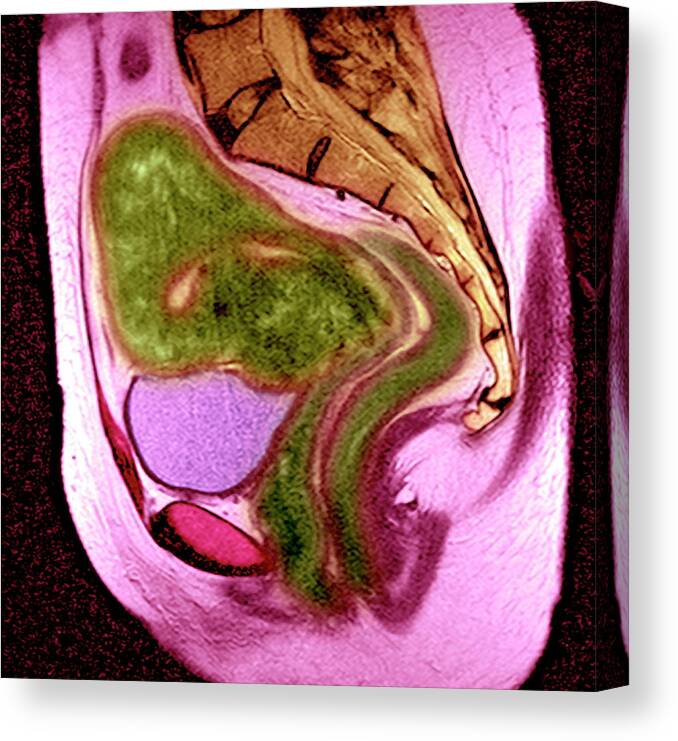The image showcases a detailed, abstract design that resembles a piece of art or a cutaway of a colorful stone. At its core, the shape is primarily oval and dominated by a bright pink exterior adorned with red lines. Within this striking frame is a green, amoeba-like figure, giving the impression of an alien baby. This central figure contains two yellow, raindrop-shaped features and is bordered beneath by a light purple semicircle with a red border, proceeding downwards to reveal twin red elements. Above the green entity, a structure mimicking a wing emerges, featuring black stripes on a brown lower section and darker brown veins on its upper part. The outer pink area exhibits a scaly texture and the entire composition is flanked by darker brown shades on both sides, further enhancing the visual complexity. The abstract nature of the design could evoke interpretations ranging from a stylized medical sonogram to a fantastical representation of a distorted x-ray, although the vivid, non-realistic colors add to the ambiguity.